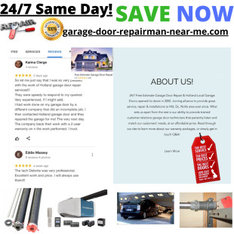The image primarily features a promotional ad with a predominantly white background on the top left, transitioning to black and bold on the right side, where the text "24/7 Same Day" is underlined. Prominent green text declares "SAVE," followed by "NOW" in blue, with "garage-door-repair-near-me.com" highlighted brightly beneath.

Upon closer inspection, the left side of the image reveals a blurry depiction of a house, seemingly painted in a grayish-blue hue. There appear to be review symbols, possibly five stars with accompanying comments, but they are too blurred to decipher. Black font lines across various sections of the image are similarly illegible. There is also a light blue rectangle, with "About Us" written in black, although this section, too, is unclear.

Additionally, a red tag with white text stands out, yet is unreadable. Within the blurred backdrop, a black car is visible along with grayish pipes, set against a beige wall. Other vaguely gray and teal elements hint at further details, but remain indiscernible due to the image’s lack of clarity.